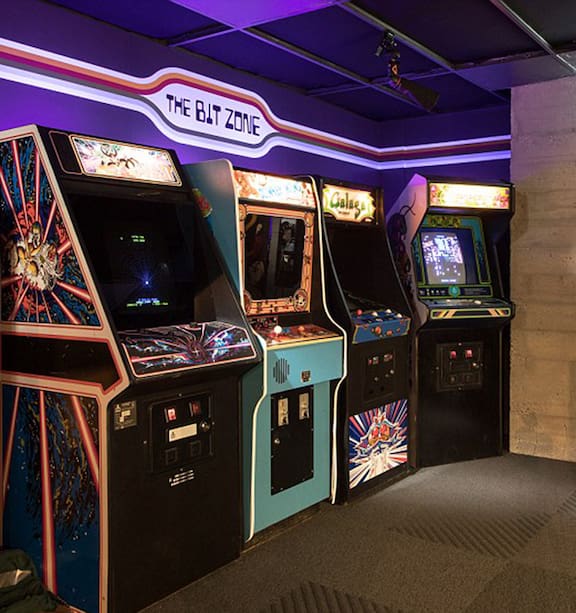The image captures an indoor arcade room illuminated by a glowing pink ceiling light, casting a nostalgic ambiance reminiscent of the late 1980s. The arcade features a gray, big-squared carpeted floor with textured patterned tan blocks adding some depth and color variation, extending to a wooden wall or door on the right. Dominating the scene are four vintage stand-up arcade machines—all positioned against a purple wall. Each machine has its characteristic joystick and retro monitor, ready to transport players back in time. Notable among them is a Galaga machine, positioned third from the left, while another machine hints at being Ms. Pac-Man. Each arcade cabinet sports a different color scheme: black, teal blue, dark blue with orange sides, and another black. Above these machines, an illuminated sign that reads "The Bit Zone" (with some ambiguity in the exact name) stands out with its intricate borders—white, then red, followed by purple—adding a bright, inviting allure to the space. Though no people are present, the room's glowing lights and classic décor vividly capture the nostalgia of an 80s gaming haven.